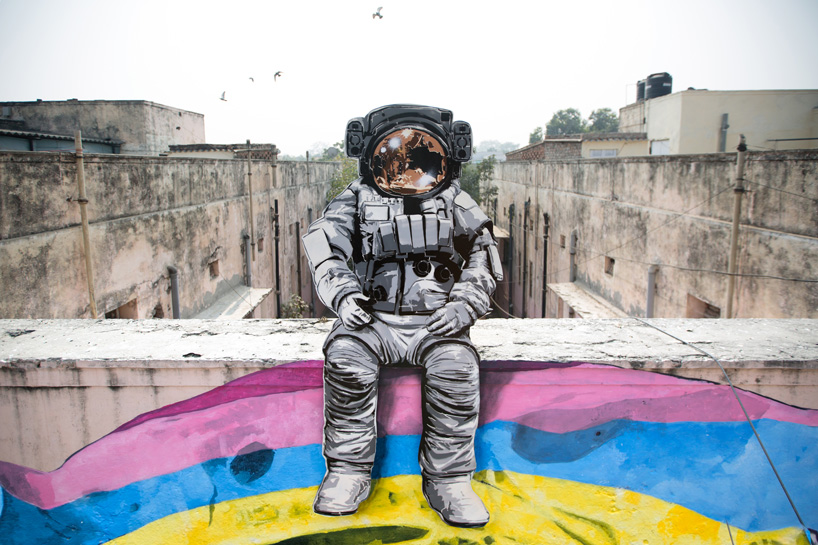The photograph depicts an astronaut sitting on a white marble wall or ledge, which serves as a connection between two interconnected, U-shaped, stone or concrete buildings. The architecture in the background evokes a bleak, industrial, communist-era aesthetic, devoid of color and teeming with decay. There are four birds soaring in the gray, unadorned sky above the scene, adding a touch of life to the somber setting. The astronaut is garbed in a grey-to-silvery space suit adorned with black contraptions and a striking golden, orb-shaped visor complemented by a black helmet. His or her feet rest upon a vividly colored mural or banner, featuring undulating stripes of yellow, blue, red, and purple. The astronaut's hands are positioned on their legs, fully covered by thick gloves, imbuing the figure with a sense of stillness and introspection as they gaze ahead, their visage obscured by the reflective helmet.